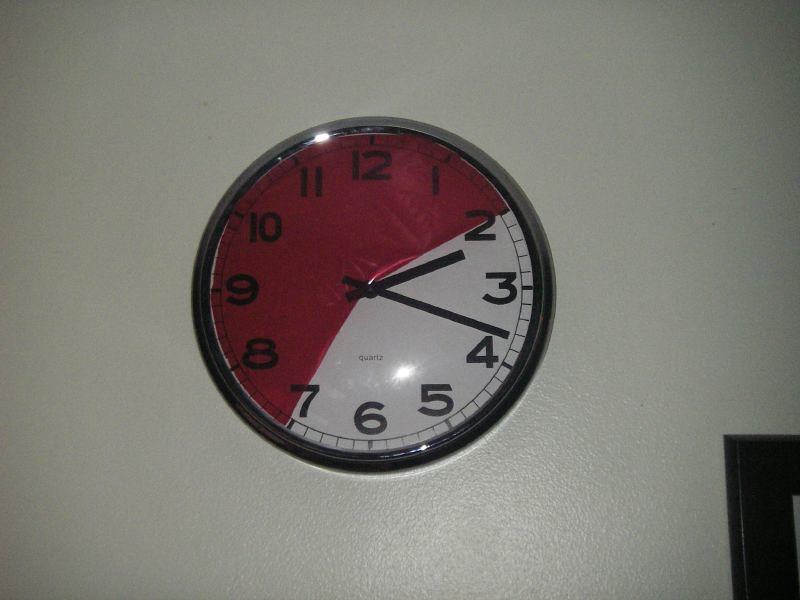This image features a round wall clock mounted on a white wall. The clock is framed by a sleek, chrome border approximately half an inch to an inch thick. The clock face is primarily red, but a segment from the 2 o'clock position to the 7 o'clock position is white, creating a striking contrast. The time displayed on the clock is around 2:17 or 2:18, indicated by black rectangular hour and minute hands. The clock face is adorned with black Arabic numerals, clearly marking each hour. The reason for the color division on the clock face is not immediately apparent.